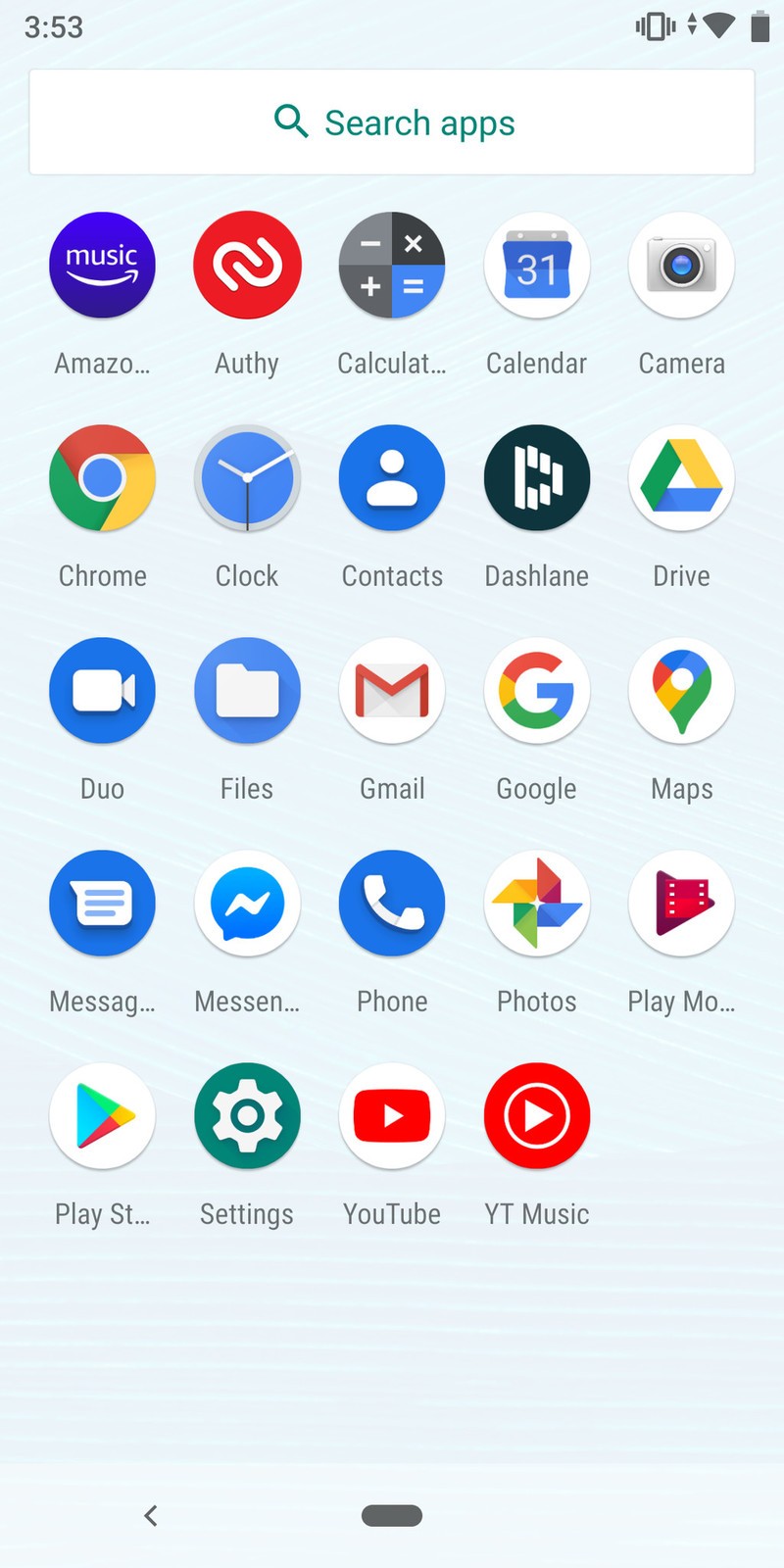The image depicts a cell phone screen with a variety of elements. In the upper left corner, the number "353" is displayed, while the upper right corner shows status indicators for "vibrate," signal bars, Wi-Fi, and a full battery. Below these indicators is a white and green search bar with a magnifying glass icon and the text "Search apps" on a white background. 

The main section of the screen features a grid layout consisting of five rows and five columns of app icons. 

- The top row includes:
  1. Amazon Music 
  2. Authy 
  3. Calculator 
  4. Calendar
  5. Camera
  
- The second row includes:
  1. Chrome
  2. Clock
  3. Contacts
  4. Dashlane
  5. Drive
   
- The third row includes:
  1. Duo
  2. Files
  3. Gmail
  4. Google
  5. Maps

- The fourth row includes:
  1. Messages
  2. Messenger
  3. Phone
  4. Photos
  5. Play Store (abbreviated as Play S-T...)

- The fifth row includes:
  1. Settings
  2. YouTube
  3. YT Music 

The dominant colors of the icons are blue, red, yellow, and green, while the phone itself appears in shades of gray, black, and white.